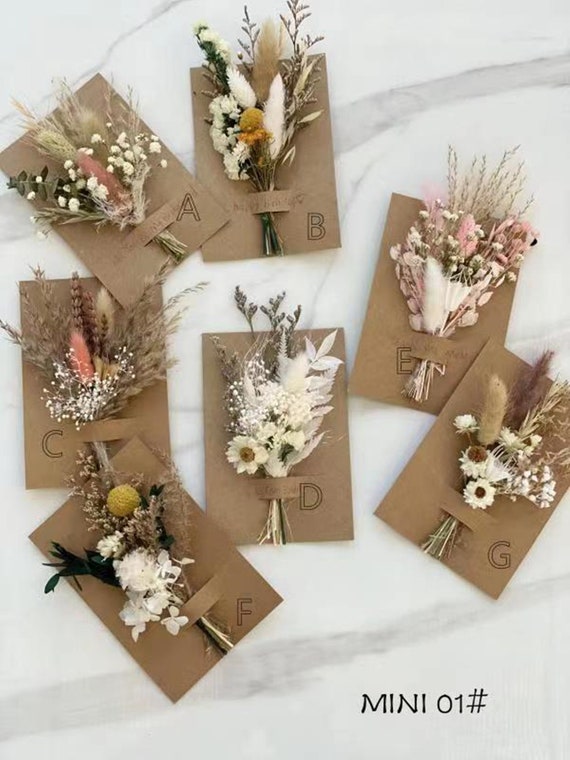This image showcases seven small dried flower arrangements meticulously positioned on a brown cardboard background. Each arrangement is labeled sequentially from A to G. The flowers display a variety of colors: 

- Arrangement A features white and yellow flowers interspersed with greenery.
- Arrangement B consists of delicate pink flowers along with green accents.
- Arrangement C combines brown and pink flowers, accented with green foliage.
- Arrangement D, positioned centrally, is a predominantly all-white arrangement with a prominent daisy that boasts a vibrant yellow center.
- Arrangement E, identical in label to D, also contains a blend of white and pink flowers mixed with greens.
- Arrangement F stands out with a striking yellow ball atop, complemented by black feathers and white flowers in the foreground.
- Lastly, Arrangement G mixes tan, white, and brown flowers, again interspersed with green elements.

These miniature arrangements bear an uncanny resemblance to magnified boutonnieres. At the bottom of the arrangement display, the text "Mini 01 #" is printed in black against a white background, adding a formal label to the scene.